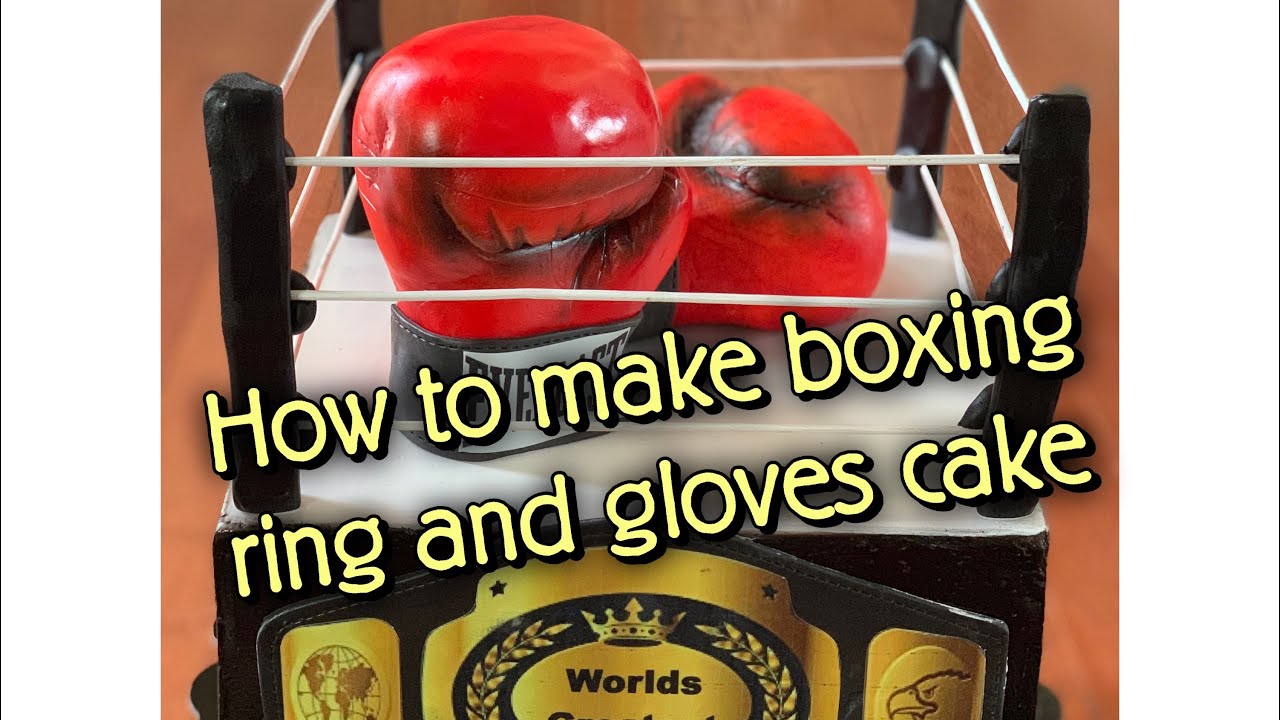The detailed and descriptive caption for the image, combining shared and repeated elements from all three submissions, would be:

"This is a highly detailed photograph of an elaborate cake, designed to resemble a miniature boxing ring complete with red fondant boxing gloves at the center. The cake's base features a meticulously crafted gold and black heavyweight championship belt adorned with an Earth emblem, laurel rings, a crown, and an eagle, although part of the belt’s inscription appears cut off, it reads 'worlds' clearly. The boxing ring itself is black and white, with three ropes strung along all four sides of the ring from post to post. The gloves, positioned upright in the center, are slightly weathered and branded with what looks like 'Everlast' on the wrist. The background of the image is light orange, but unclear. Across the middle of the photo, the caption reads, 'how to make boxing ring and gloves cake.'"